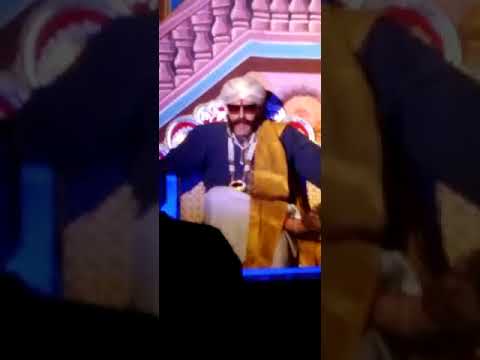This image, likely a screenshot from a movie scene or possibly a computer-generated image, depicts a well-dressed man seated on an ornately decorated throne. The man, who appears to have Eastern Indian features, dons a blue button-down silk robe coupled with numerous pieces of jewelry and a golden yellow sash draped over his left shoulder. Sporting thick, bold mustache and sideburns, he also wears square sunglasses and a turban, adding to his distinguished and regal appearance. The throne he sits on features a red backrest with gold accents and a potentially blue and yellow bottom section. Behind him, a staircase, which appears artificial, ascends with purple columns and blue and red lines at the base. The poorly lit and somewhat blurry quality makes it challenging to discern every detail, though it seems as though there might be another figure partially in the frame, casting a shadow that blocks a part of the man on the throne. The overall setting suggests an indoor environment and the image carries an impression consistent with an extravagant Bollywood film scene.